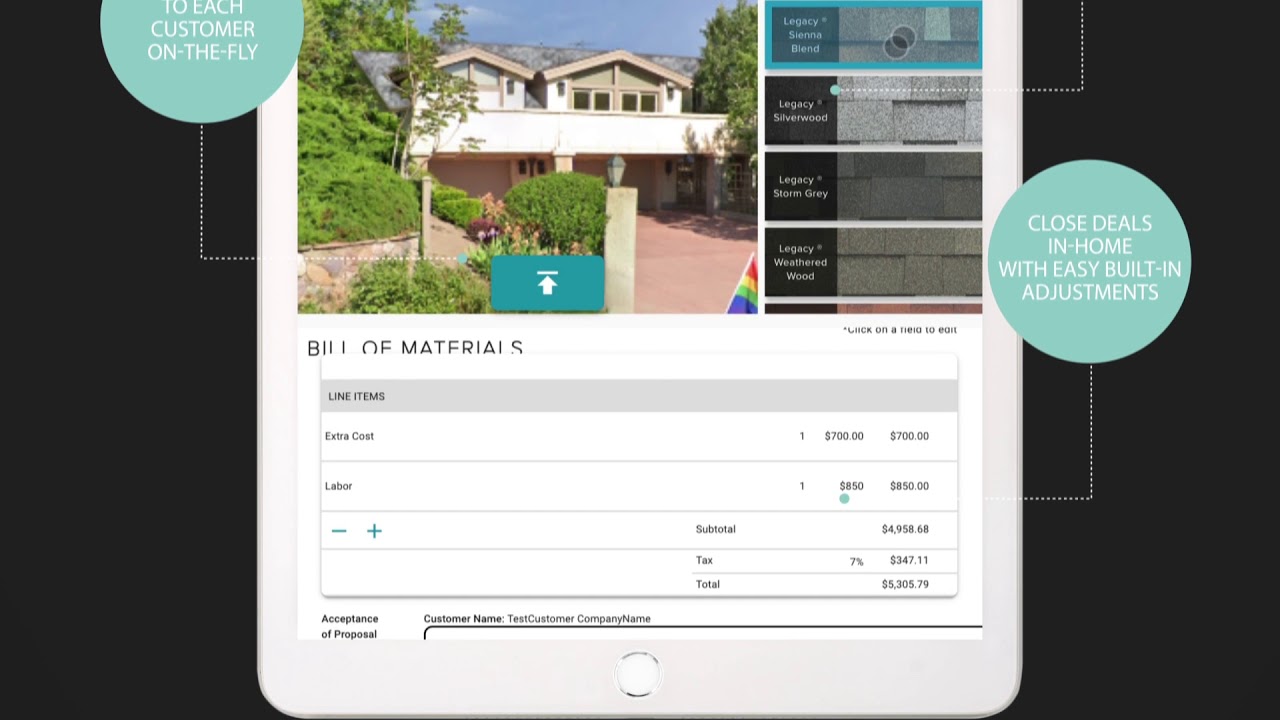A detailed, cleaned-up caption for the image might look like this:

"This image, sourced from a website, features a central graphic of a white smartphone set against a black background. At the top of the smartphone screen, there is a photograph showing a house surrounded by lush green trees and bushes. Adjacent to this image, the text 'Legacy Blend' appears, indicating selections of roofing options. Labels such as 'Legacy Storm Grade' and 'Weathered Wood' are listed as possible choices.

Below these options, there is a detailed billing section. It includes line items such as materials and labor, with respective costs listed: extras costing $700 and labor at $850, leading to a subtotal of $4,958.68. With an added tax of $347, the grand total amounts to $5,305.79. 

Flanking the smartphone graphic are light blue circular icons. The one on the left reads 'Teach customers on the fly', while the one on the right states 'Close details in-home with easy built-in adjustments'."